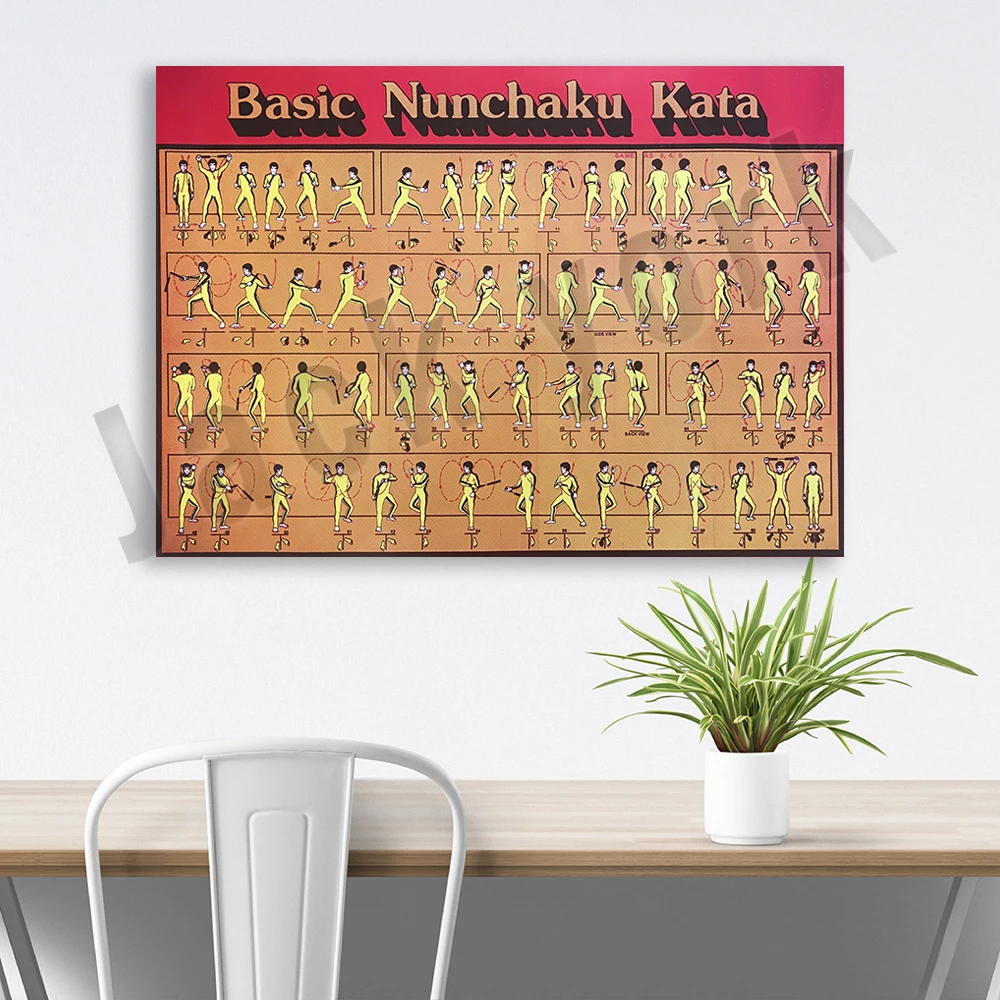A visually striking poster titled "Basic Nunchaku Kata" is centered on a pristine white wall. Surrounding the poster below is a light brown wooden countertop that houses a white planter with a vibrant green plant. In front of the countertop, a white metal chair is positioned neatly. 

The poster itself stands out with its bold red top section, featuring the title in light brown letters, accented by a black shadow effect. Arranged in four distinct rows, the poster showcases animated sequences of a man dressed in a yellow suit with black hair. He is dynamically demonstrating various nunchaku techniques, with red arrows indicating the movement paths and diagrams specifying his foot positions for precision. Each character illustration vividly captures different stances and actions, making the poster both instructional and engaging. The scene is completed by the clean and orderly appearance of the area, creating an inviting and organized atmosphere.